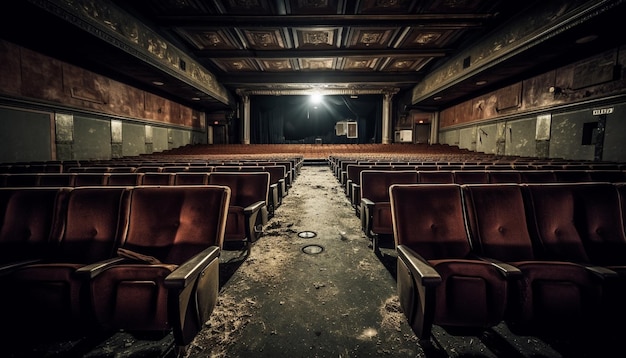The photograph captures the forlorn beauty of an abandoned movie theater, viewed from the front row, looking down a dusty aisle lined with rows of plush seats. The atmosphere is steeped in darkness, except for the distant glow of the projector's light at the very back, casting an eerie illumination. The seats, once luxurious in hues of purple and red velvet, are now in disrepair, folded up, and dotted with debris and cobwebs. The floor is strewn with dust and sawdust-like particles. Despite the dereliction, the intricate design of the theater ceiling offers a glimpse into its former grandeur, though now shrouded in shadow. The theater exudes a haunting ambiance, silent and vacant, as if time had forgotten this once vibrant place.